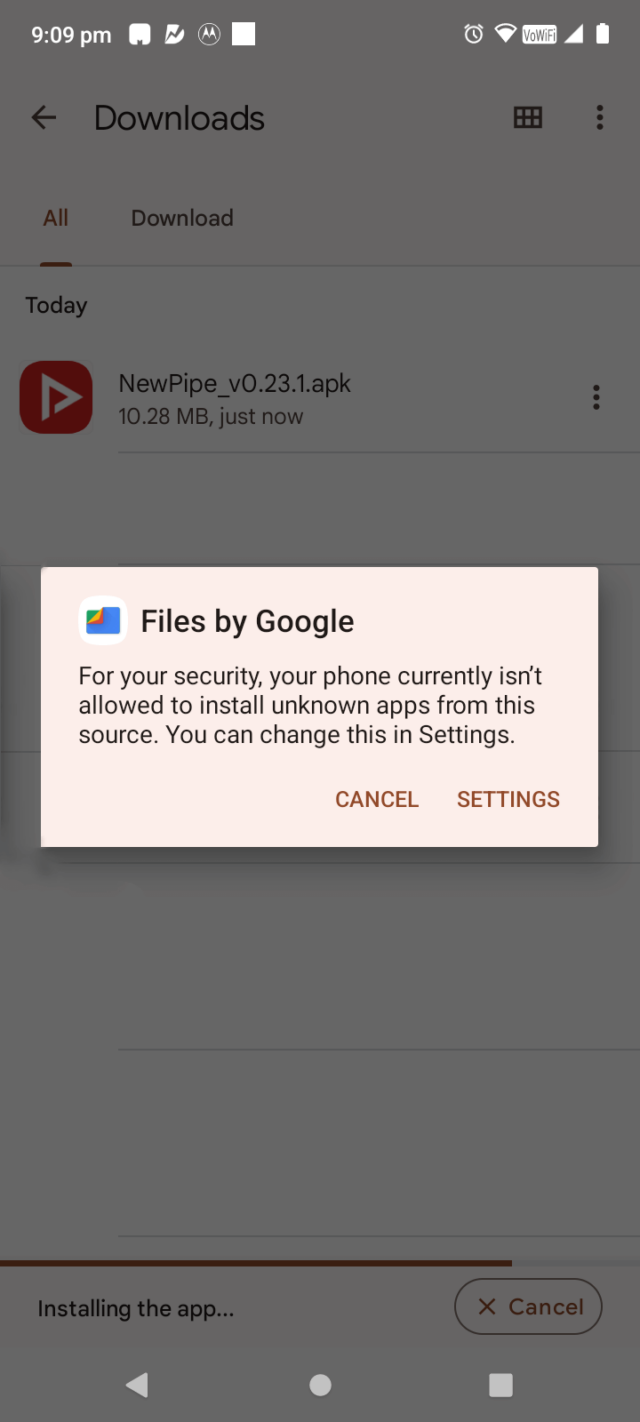**Detailed Image Caption:**

The image is a screenshot of the download section on an Android phone, captured at 9:09 AM. At the top of the screen, several status icons are visible. Starting from the left, there are a few unidentified icons, including one that features a zigzag inside a "D". This is followed by the Motorola logo, a white square icon, an alarm clock, a partially filled Wi-Fi icon, a "VO" indicator next to the Wi-Fi, a full cellular signal bar, and a fully charged battery icon.

The background of the screen is grayed out with a semi-transparent overlay dialog on top. The main background portion shows the "Downloads" section, featuring a back arrow on the upper left. Below this are two tabs "All" and "Download options", with "All" being selected in red. Under the "All" tab, a download list is visible, starting with "Today". There is a red and white triangular download icon next to a file named "newpipe_V0.23.1 APK" which is 10.28 megabytes in size and listed as "just now".

Over the grayed-out background, a pop-up window from "Files by Google" is displayed, indicating a security alert. It states, "For your security, your phone currently isn't allowed to install unknown apps from this source." Below this message are two text buttons: "CANCEL" on the left and "SETTINGS" on the right. Directly above this alert, another pop-up showcases the "Installing" progress of the app, which appears to be approximately 80% complete, with a "CANCEL" button located at the lower right corner of this installation progress dialog.